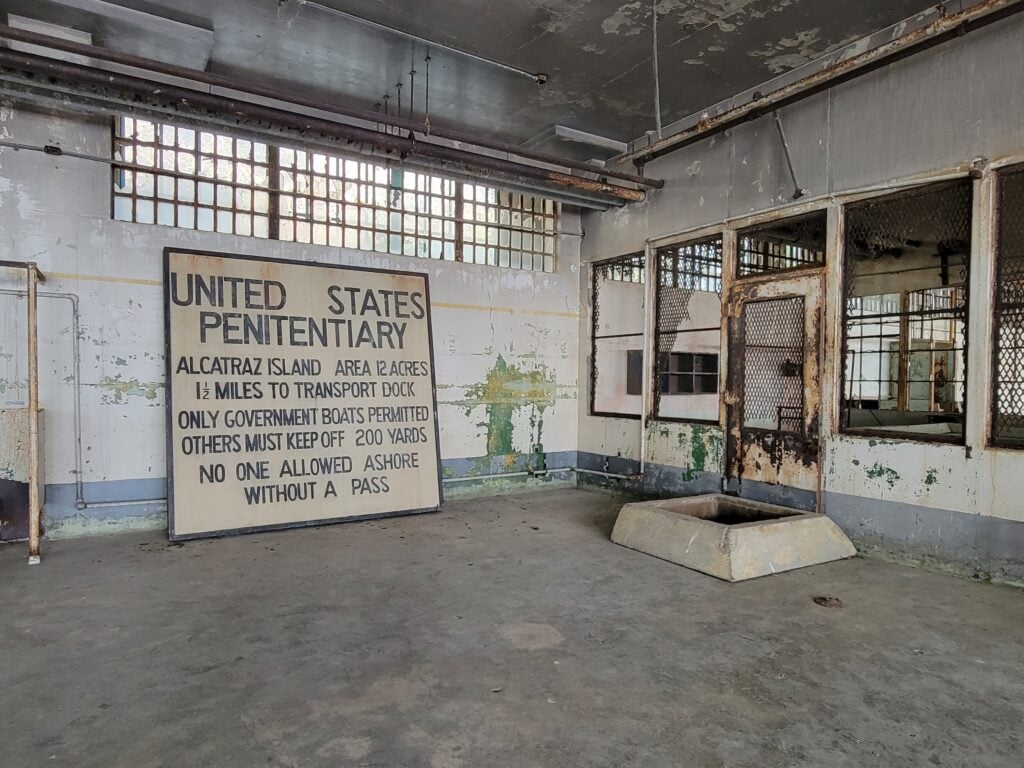This photograph captures the stark interior of a room in Alcatraz prison, characterized by its dreary, off-white cement walls with peeling paint and signs of mold, and a metal ceiling. The room's concrete floor adds to its cold, barren atmosphere. Exposed pipes run along the ceiling, enhancing the industrial feel. On the far wall, leaning precariously, is a large, yellowed sign with a black border, almost reaching halfway up the wall. The windows above the sign are barred and rusted, with some of the metal mesh having broken away, likely due to the corrosive salty air. The prominent text on the sign reads, "United States Penitentiary," followed by "Alcatraz Island Area, 12 acres, one and a half miles to transport dock, only government boats permitted, others must keep off 200 yards, no one allowed ashore without a pass." The right side of the room features a rusty, caged door, indicative of years of neglect and exposure to the elements. This detailed image reflects the harsh, decaying environment of the infamous Alcatraz prison near San Francisco.